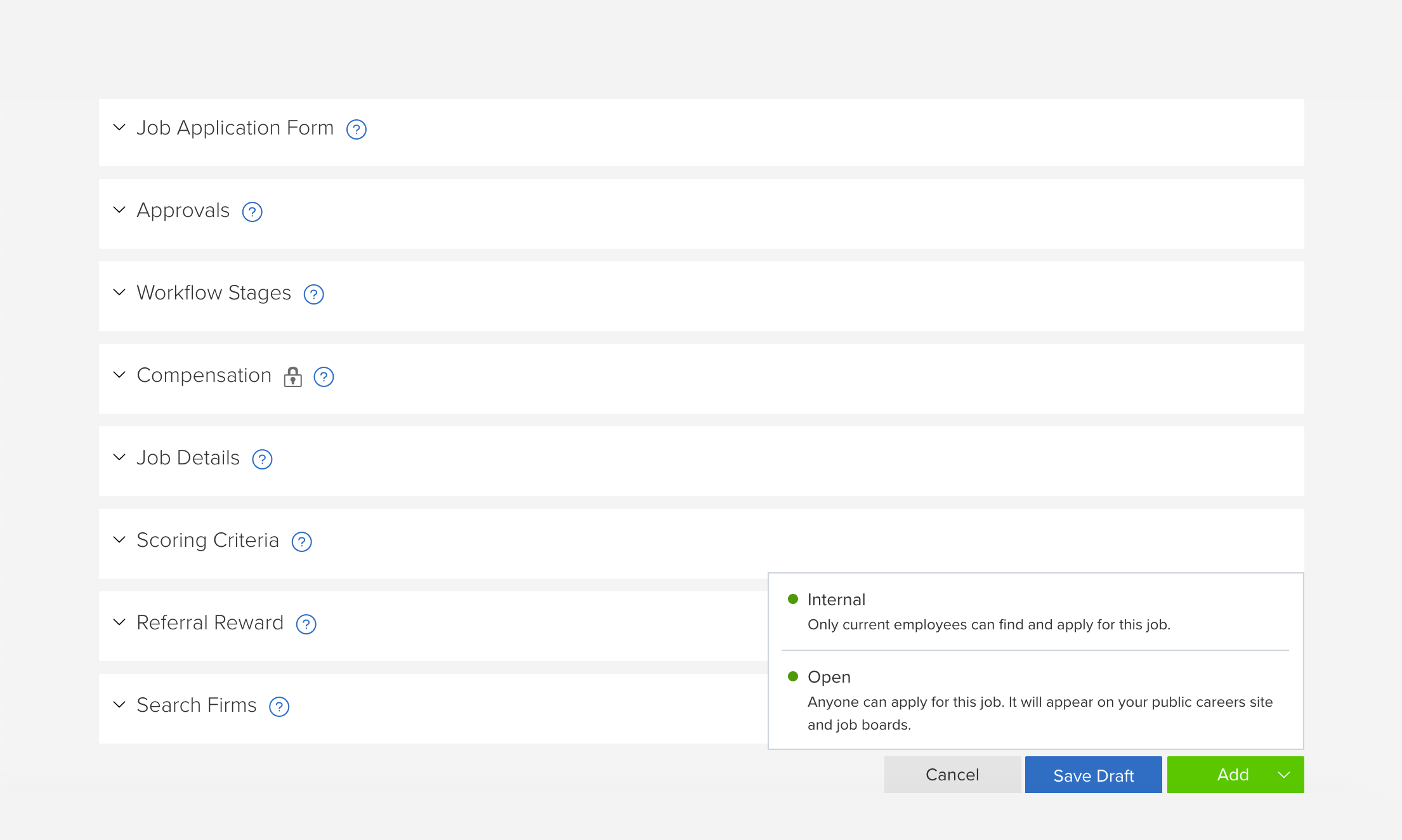This image showcases a user interface featuring a job application management system. The background is a subtle gray, contrasting with the white backdrop of multiple drop-down menus. There are eight drop-down menus aligned vertically from the top left corner, each associated with a specific stage or detail of the job application process. The titles of these menus are as follows: "Job Application Form," "Approval," "Workflow Stages," "Compensation" (marked with a lock icon), "Job Details," "Scoring Criteria," "Referral or Reward," and "Search Firms." At the end of each title is a blue circle containing a white question mark, serving as a help icon.

On the bottom right side of the interface, there are two descriptions accompanied by green dots. The first description states, "Internet Only: Current employees can find and apply for this job." The second description reads, "Open: Anyone can apply for this job. It will appear on your public career sites and job boards."

Below these descriptions, three buttons are positioned at the bottom right corner of the interface. "Cancel," identified by its gray color; "Save Draft," distinguished by its blue color; and "Save & Continue," highlighted in green. These buttons provide the user with options to cancel the process, save their progress as a draft, or proceed with saving and continuing to the next step.